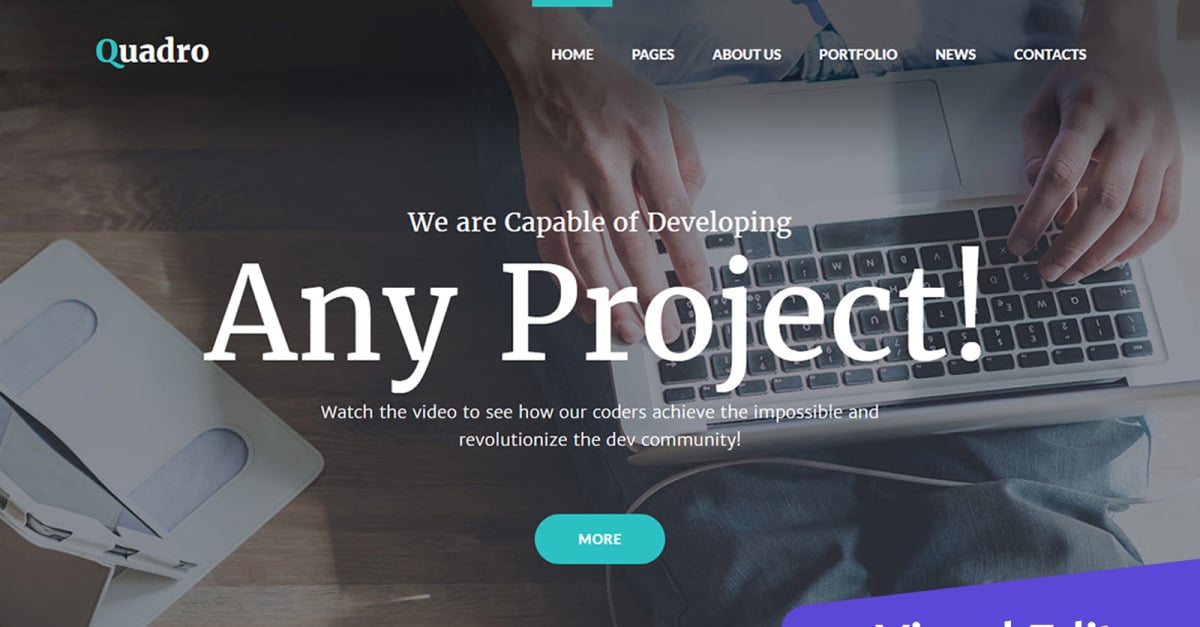In the screenshot, a man is seated on a wooden floor with his laptop resting on his lap. The laptop screen displays a website under the brand name "QUADRO," highlighted by its distinctive blue 'Q' and white lettering for the remaining characters. The website's navigation bar lists several sections: HOME (underlined with a blue line), PAGES, ABOUT US, PORTFOLIO, NEWS, and CONTACTS. Beneath the navigation bar, there is a prominent message that reads, "We are capable of developing any project!" urging viewers to watch a video that demonstrates how their coders achieve groundbreaking feats that revolutionize the development community. Additionally, the website features a section labeled "DEV," marked within a green oval with the word "more" in white text inside it. Towards the bottom of the screen is a partially visible purple oval containing more illegible white text.